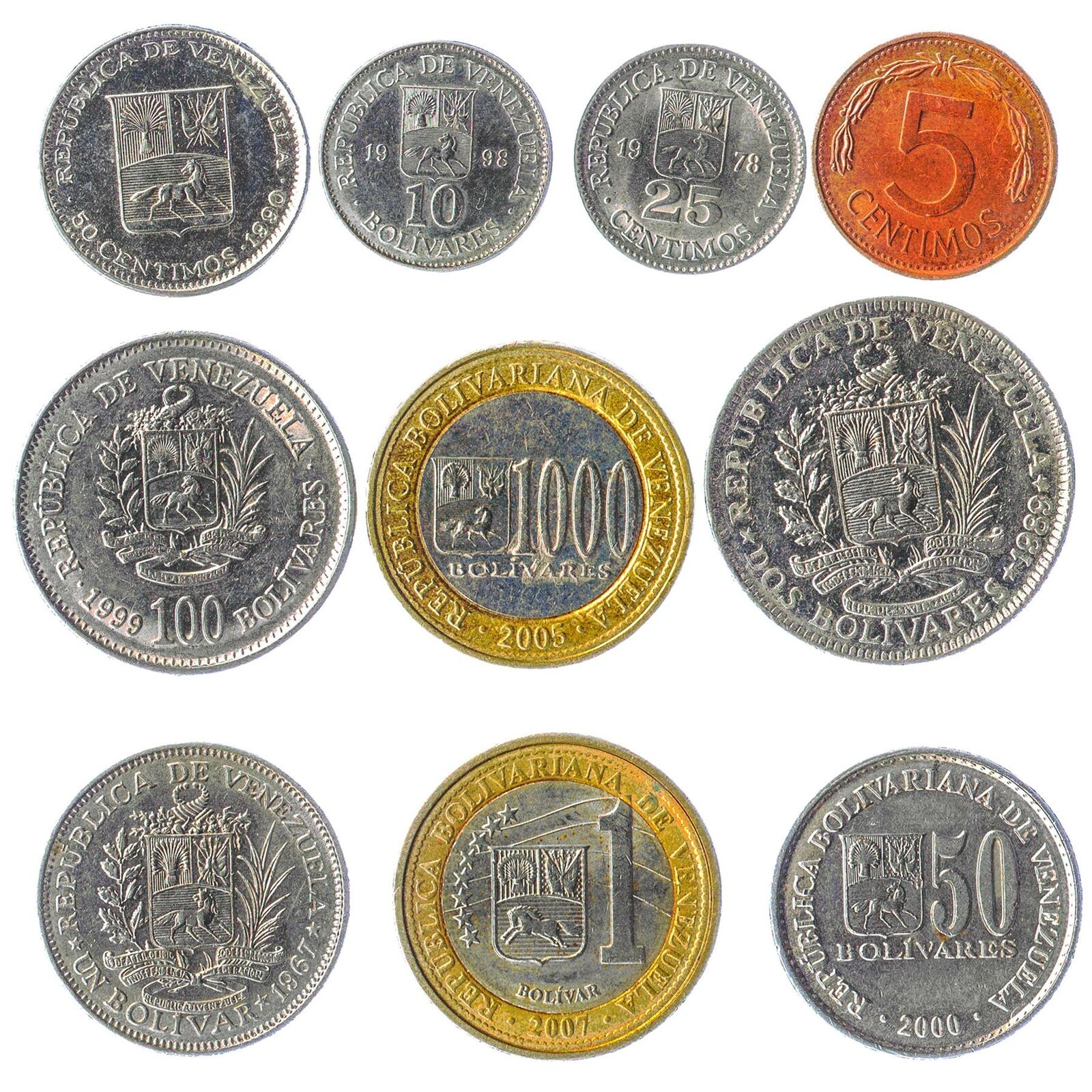The image showcases a collection of Venezuelan coins set against a pure white background, featuring a square layout without visible borders. The top row displays four coins: three silver and one copper-colored, progressing from left to right. Specifically, there is a 50 centimos coin from 1990, a 10 bolivars coin from 1998, a 25 centimos coin from 1978, and a copper 5 centimos coin. Below the top row, there are two rows, each containing three larger coins. These middle and bottom rows include silver coins ringed in gold with various designs and denominations, such as 100 bolivars from 1999, 1,000 bolivars from 2005, and 50 bolivars from 2000. The coins showcase a broad range of dates from 1867 to 2007, with inscriptions in Spanish and values indicated as centimos and bolivars. Notable features include shields and other etched designs, emphasizing their diverse denominations from one bolivar to 1,000 bolivars, and their historical spread.